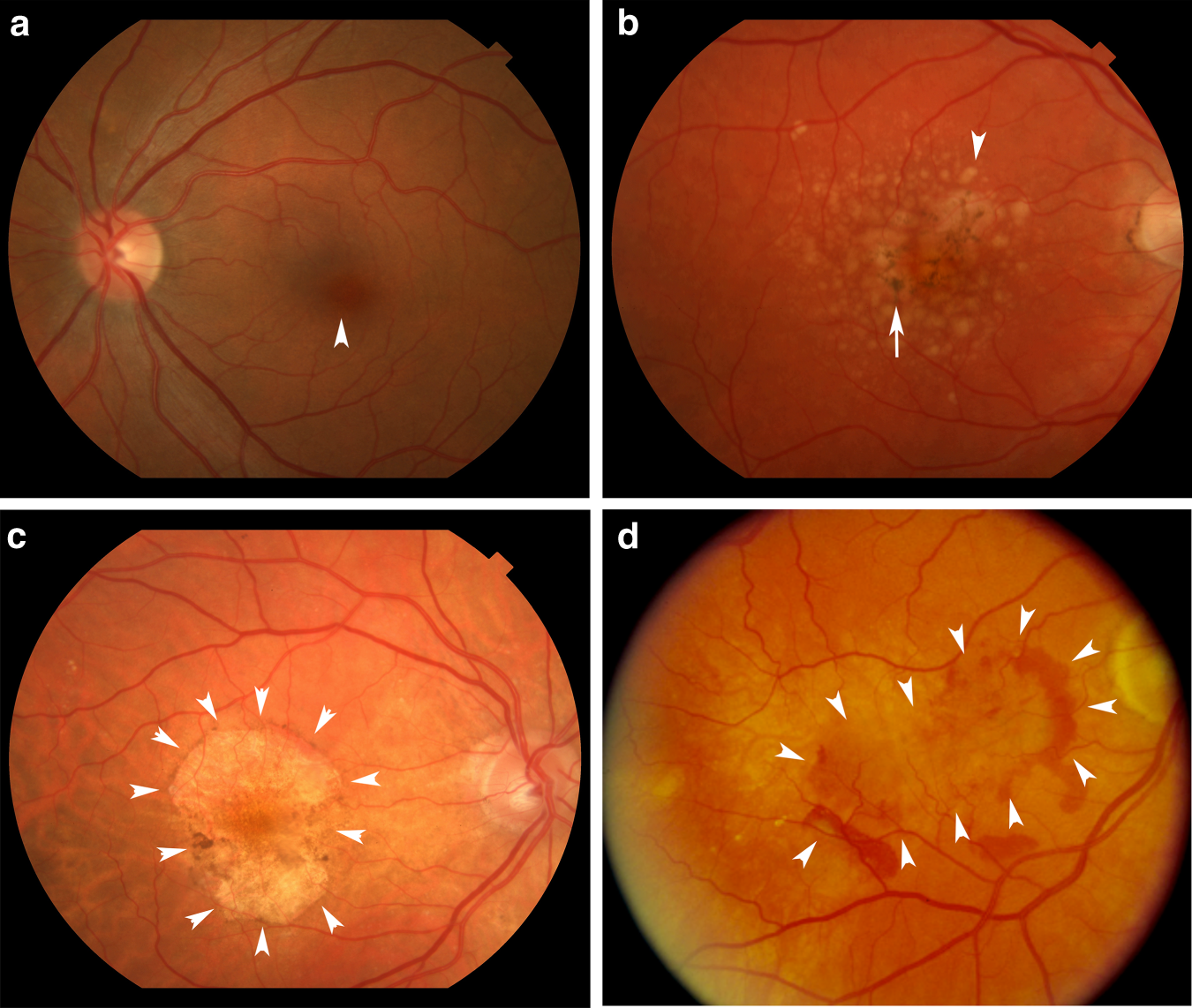This set comprises four detailed retinal images labeled A, B, C, and D. The images are organized with A and B on the top row and C and D on the bottom row. Each circular photograph captures different views of the retina, featuring a prominent yellowish-reddish coloration interlaced with an intricate network of veins, all set against a dark background.

- **Image A (Top Left)**: This image highlights the central spherical structure of the retina, with branching veins permeating outward. Near the middle of the image, a small white arrow indicates a darker, bruise-like area, drawing attention to a specific region of potential concern.
  
- **Image B (Top Right)**: Two arrows are present in this image. The central arrow points upwards towards a small black dot, while a second arrow above it, pointing downwards and slightly to the right, directs attention to another, less distinct area.
  
- **Image C (Bottom Left)**: A lighter, roundish area stands out in this image, marked by a total of eleven small arrows converging on this single spot. This clustering of arrows suggests a significant focal point within the retinal landscape.
  
- **Image D (Bottom Right)**: Unlike the more circular area in Image C, this view shows an oblong shape similarly highlighted by an array of twelve arrows pointing towards it. The arrows collectively emphasize another critical region within the retina.

These images collectively offer a comprehensive examination of the retina, with each annotated element guiding viewers to specific areas of interest or potential pathology.